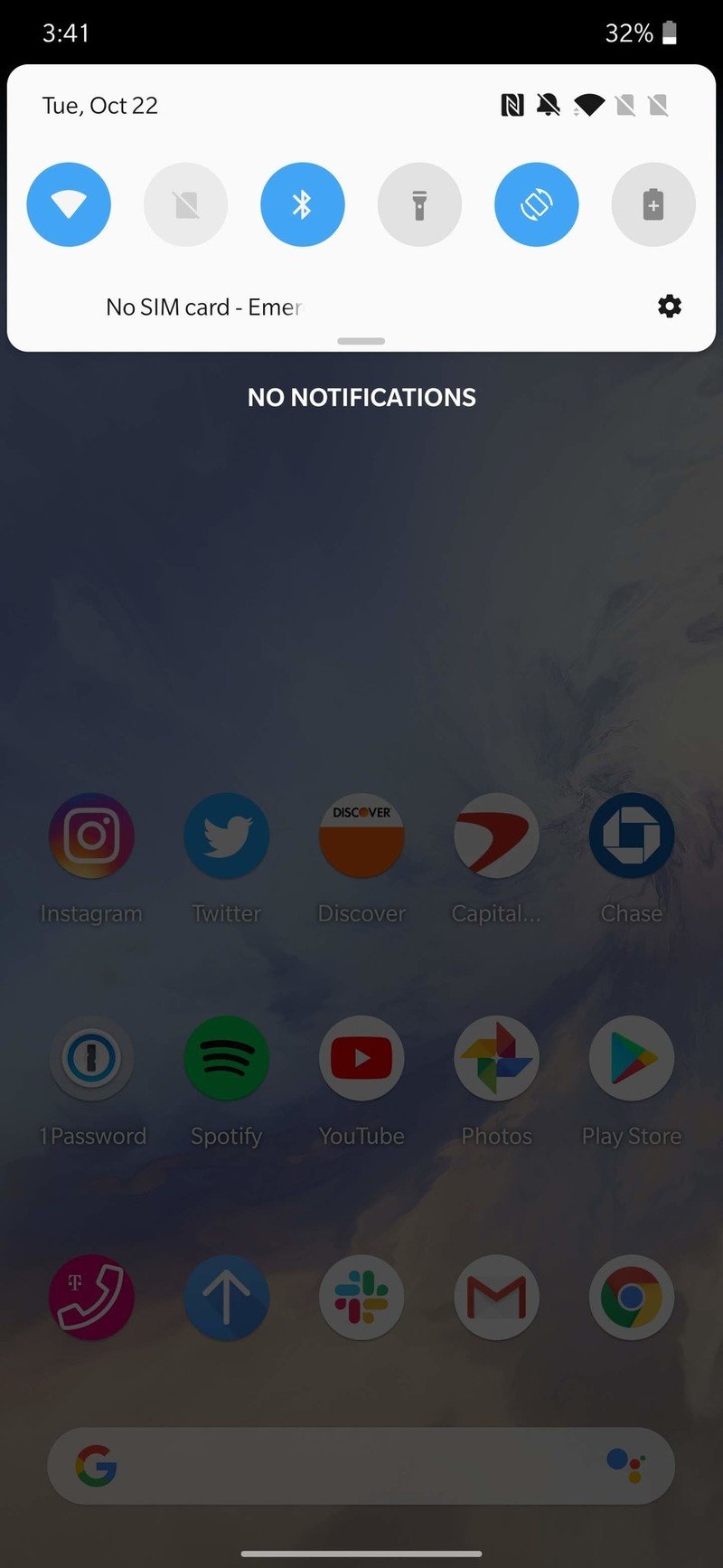The image is a detailed screenshot of a smartphone home screen. At the very top, there is a black border, showing the time as 3:41 on the left, though it does not specify AM or PM. On the right side of this border, the battery icon indicates a charge level of 32%. Directly below, a white rectangle with rounded corners displays the date, "Tuesday, October 22nd."

Beneath the date, there are several icons in alternating blue and gray circles. The Wi-Fi and Bluetooth icons are white against a blue background, whereas the battery and flashlight icons are against a gray background. Additionally, it displays a message, "No SIM card," followed by a dash and the partial word "EMER," likely indicating "Emergency."

The background is dimmed, suggesting a pop-up menu is active, which contains a white text notification stating "No notifications."

As the main content, the home screen displays three rows of app icons, including popular applications such as Instagram, Twitter, Capital One, Chase Bank, Spotify, YouTube, Google Photos, Google Play, Gmail, and Chrome. At the very bottom of the screen, there is another white rectangle with rounded corners, serving as the search box for the Google app.